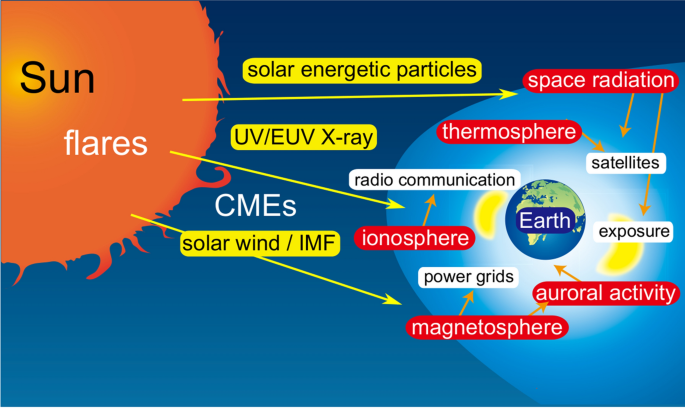The image is a detailed color diagram depicting the interaction between the Sun and the Earth, highlighting various scientific phenomena. The background is blue, and on the upper left corner, there is a large orange circle representing the Sun, labeled "Sun" in black text with "Flares" in white text nearby. Flames or solar flares are emanating from the Sun. From the Sun, three yellow arrows point towards the Earth, labeled "Solar Energetic Particles," "UV/EUV X-ray," and "Solar Wind/IMF." Above these, the term "CMEs" (Coronal Mass Ejections) is mentioned.

On the right side of the diagram is a smaller, round blue Earth with green land masses, labeled "Earth" in white text, surrounded by a lighter blue background that extends from the right side. Around the Earth are multiple labeled elements and arrows indicating their effects:

- "Solar Energetic Particles" connects to "Space Radiation," which further connects to "Satellites" and "Exposure."
- "Thermosphere" also points to "Satellites."
- "UV/EUV X-ray" points to "Ionosphere," which in turn points to "Radio Communications."
- "Solar Wind/IMF" points to "Magnetosphere," connecting to "Power Grids."
- "Magnetosphere" also points to "Auroral Activity," which is associated with the Earth itself.

The diagram comprehensively illustrates how solar phenomena impact various aspects of Earth's environment and technological infrastructure, including radiation exposure, satellite operations, power grids, and radio communications.